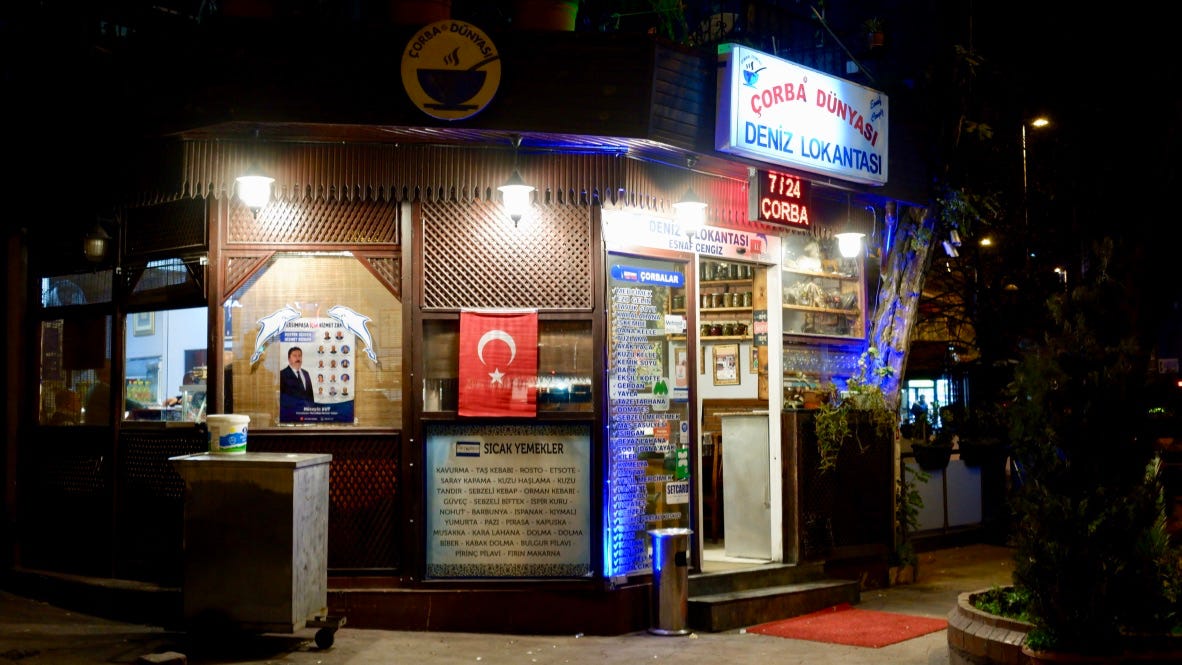This nighttime photograph captures the exterior of a small, corner eatery likely located in Turkey. The establishment, named "Korba Dunyasi Deniz Lokantasi," features a wooden facade with an illuminated sign indicating it is open 24/7, with "724 Korba" prominently displayed. Hanging from one of the windows is a red Turkish flag adorned with a crescent moon and a star. The entrance, located to the right, is open, offering a glimpse of various goods inside. The cafe is situated on a city street, flanked by other buildings with small windows, illuminated by streetlights. The setting includes an orange welcome mat, a sidewalk, and a few plants, adding to the cozy nighttime ambiance.